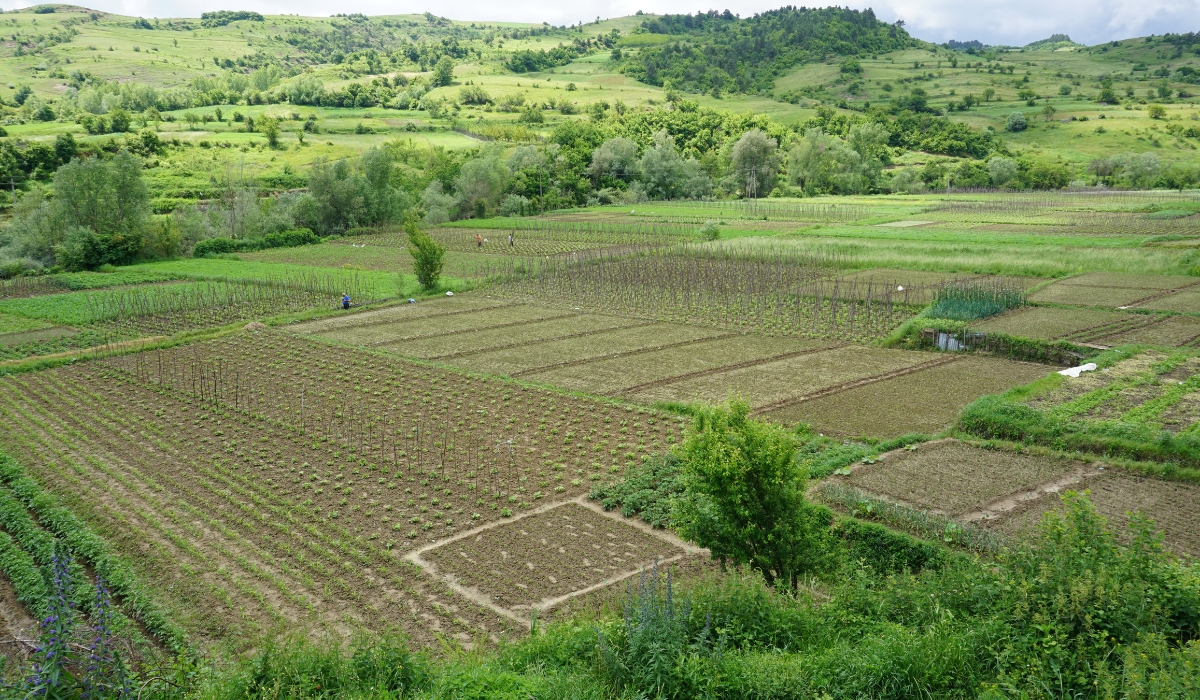This photograph captures a sprawling farmland with a patchwork of meticulously organized garden plots interspersed across the verdant landscape. The plots range from small squares to longer rectangles, each hosting diverse crops arranged in distinct rows, though their specific types are indiscernible. The scene is dotted with small trees and bushes, creating a harmonious blend of cultivated land and natural greenery. In the background, rolling hills extend towards a horizon peppered with trees and open grasslands, giving way to a lightly clouded, bluish-gray sky visible in the top right corner, suggesting a cloudy day.

Three individuals can be seen in the image: one appears to be kneeling and dressed in blue, while the other two are standing, one in red and the other in white. These figures provide a sense of scale to the vastness of the farmland. The combination of meticulously plotted land, diverse crops, and the surrounding natural backdrop suggests this is a large, well-maintained farm or a substantial garden area, possibly featuring specific sections for different crops akin to a vineyard or winery. Additionally, there are scattered puddles indicating recent rain, adding to the farm's lush appearance.